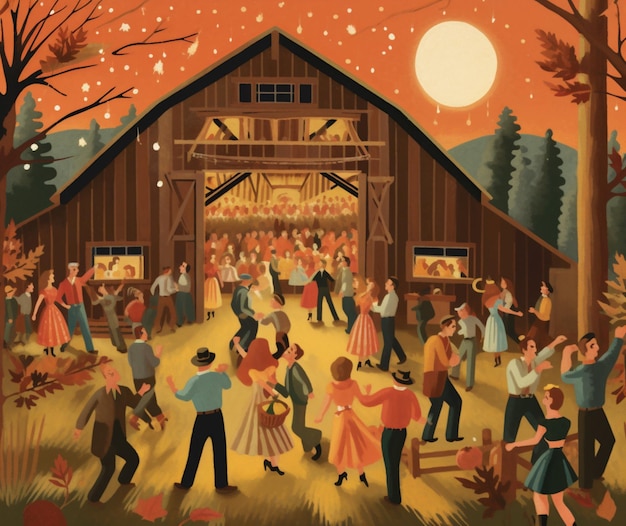This cartoonish digital drawing depicts a lively autumn festival or barn hoedown, set against the backdrop of an orange sky dominated by a large, full yellow moon and scattered yellow stars. The image, approximately four inches square, captures a vibrant scene centered on a triangular-shaped brown wooden barn, which is brimming with people celebrating and dancing. A luminous yellow light emanates from the barn's large square opening and two smaller windows, illustrating the festivity within. In the foreground, men in shirts and jackets and women in dresses dance on the light yellow grass-field outside the barn. Surrounding the barn, the mix of mostly barren brown trees with sparse dark orange and brown leaves, and the dense clusters of green and bluish-green coniferous trees in the background, encapsulate the transitional beauty of autumn. Adding to the seasonal ambiance are the occasional orange leaves and perhaps snowflakes drifting down from the sky. Distant bluish-green mountains further enrich the scenic landscape, completing the enchanting portrayal of this festive fall celebration.